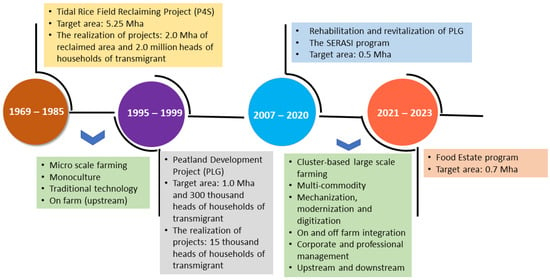The image is a detailed diagram depicting a timeline spanning from 1969 to 2023, outlining various agricultural projects and technological advancements. The timeline is divided into four main segments, each represented by circles of different colors: orange (1969-1985), purple (1995-1999), blue (2007-2020), and bright orange (2021-2023). 

Across the top, the diagram features two key project headings: a yellow rectangle on the left for the "Total Rice Field Reclaiming Project" with a target area of 5.2 MHA, realized as 2.0 MHA of reclaimed land supporting 2 million trans migrant households (1969-1985); and a blue rectangle on the right for the "Rehabilitation and Revitalization of Page 5, PLG, and CSERES Program" with a target area of 0.5 MHA (2007-2020).

The bottom of the diagram is segmented into four colored rectangles—green, gray, green, and orange—each detailing specific agricultural practices and technological milestones associated with the timeline periods. Key highlights include:
- **1969 to 1985**: Indicative phrases such as "no monoculture," "micro-scale farming," "traditional technology," and "on-farm upstream" are denoted in a green box.
- **1995 to 1999**: Focus on "Peatland Development Project" with a target area of 1.0 MHA and 300,000 trans migrant households, achieving 15,000 households.
- **2007 to 2020**: Emphasis on "Cluster-based large-scale farming," "multi-commodity mechanization," "modernization and digitization," and an "integration of corporate and professional management" both on and off the farm.
- **2021 to 2023**: Details the "Food Estate Program" targeting 0.7 MHA, contained within a tan-colored rectangle.

This comprehensive timeline vividly showcases the evolution of land development, agricultural techniques, and migrant settlement strategies over the decades.